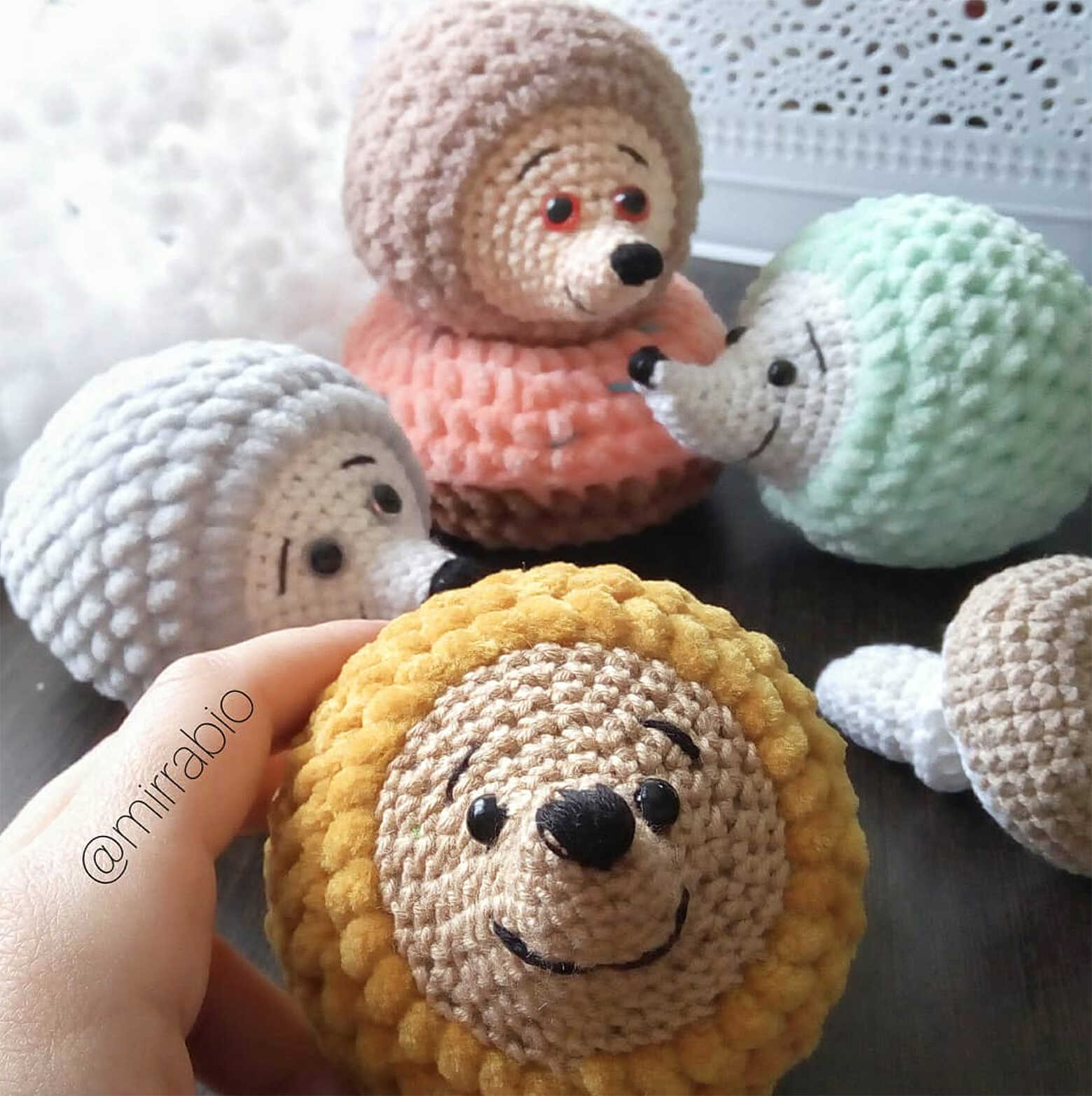This color photograph features a charming collection of knitted or crocheted hedgehogs arranged on a wooden table. At the forefront, a hand extends from the lower left quadrant, holding a yellow-furred hedgehog that faces the camera with a friendly smile. This hedgehog, along with its companions, has a brown face, black eyes, a black nose, and expressive eyebrows, which together give them a delightfully cute appearance. The hand holding the yellow hedgehog has the handle "mirabio" inscribed on one of its fingers.

In the background, three more hedgehogs are clearly visible: a white-furred one positioned directly behind the yellow hedgehog, a brown-furred hedgehog further back, and a light green (aquamarine) hedgehog towards the right. The white hedgehog has a tan face and is perched atop a pink and brown spherical object resembling a donut. Additionally, the scene includes other crocheted items such as a mushroom-like figure with a white stem and a tan cap, located near the aquamarine hedgehog. The upper right corner of the image shows a white board or grate, adding depth to the scene. This meticulously crafted, vibrant ensemble highlights the intricate details and variety of colors used in creating these adorable hedgehogs.